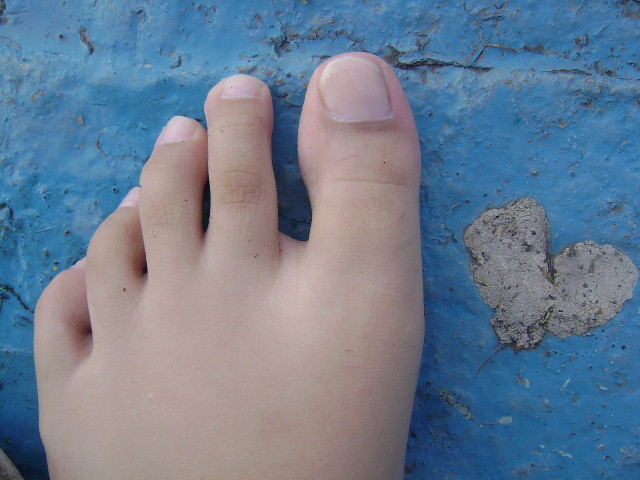This photograph captures a close-up of a small, white-skinned foot that appears to belong to a young person, possibly in middle school. The focus is on the top half of the forefoot, revealing five well-trimmed pink toenails and smooth skin. The foot, which shows a noticeable gap between the toes, rests on a blue-painted concrete surface marred by cracks and chipping paint. Specks of black dirt and gray stones are scattered across the textured ground, adding complexity to the scene. Notably, a gray heart shape is visible in the concrete to the right of the foot, providing a striking contrast to the predominantly blue background with hints of black, gray, and brown. The photo appears to be taken in an outdoor setting.